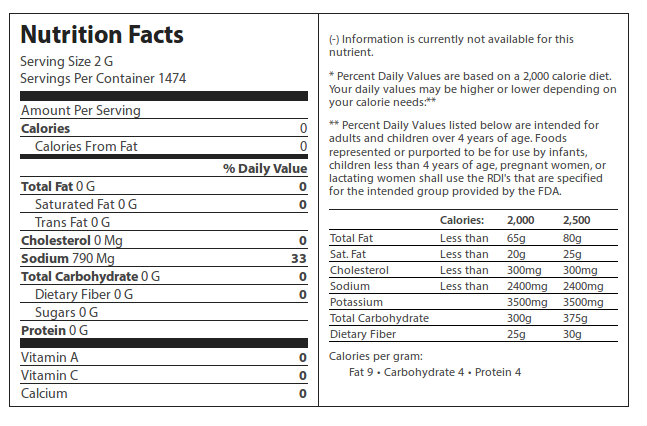The image depicts a Nutrition Facts label set against a white background with black writing. Positioned at the top in bold font is "Nutrition Facts." The label specifies that the serving size is 2 grams, and there are 1,474 servings per container. Each serving contains 0 calories, 0 grams of total fat, 0 grams of saturated fat, 0 grams of trans fat, 0 milligrams of cholesterol, 790 milligrams of sodium, 0 grams of total carbohydrates, 0 grams of dietary fiber, 0 grams of sugar, and 0 grams of protein. Additionally, it states that there are no vitamins (A, C) or calcium present. On the right section, the percentage of daily values is based on a 2,000 calorie diet. Despite the comprehensive details, the only significant component it lists is sodium, which is 33% of the daily value at 790 milligrams per serving. This suggests that the product might be an electrolyte supplement or simply salt. The image is directly posted as a digital representation, not taken from a physical object, and also includes explanatory text about what the Nutrition Facts represent.